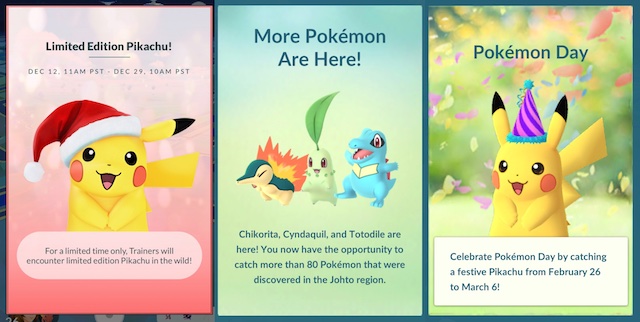This image is a promotional screenshot showcasing three different Pokémon-themed events. 

On the left, against a red background, is an image of Pikachu wearing a Santa hat. The dates "December 12th, 11 AM PST - December 29th, 10 AM PST" are displayed in gray font. The accompanying text reads, "For a limited time only, Trainers will encounter limited edition Pikachu in the wild." This indicates a special event where players can catch a festive Pikachu.

In the center section, there is a gradient background transitioning from teal blue to yellow-green. The image features three Pokémon: Chikorita, Cyndaquil, and Totodile. The text below, not contained within a box, announces, "More Pokémon are here. You now have the opportunity to catch more than 80 Pokémon that were discovered in the Johto region."

On the right, set against a purple background, is an image of Pikachu wearing a purple and dark purple party hat. The heading reads "Pokémon Day," and a white text box states, "Celebrate Pokémon Day by catching a festive Pikachu from February 26th to March 6th."

Each section highlights a unique event, offering Trainers various opportunities to catch special edition Pokémon.